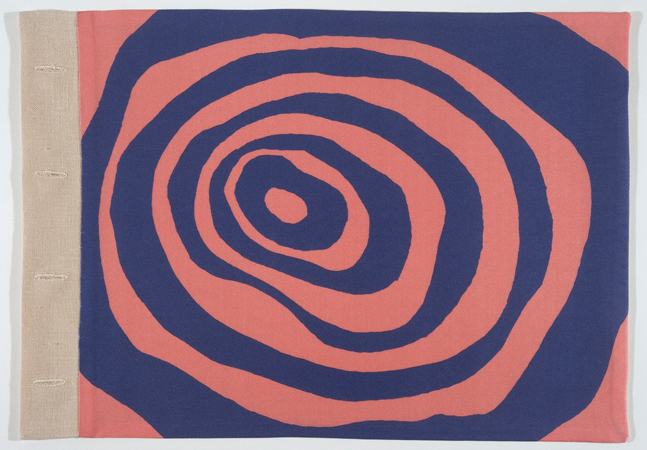This photograph features a detailed and intricate design laid against a light gray background. On the left side of the frame, there is a prominent section of burlap fabric, identifiable by its light brown color and four slits that suggest it might be threaded with a bar or string. The main design, centrally placed, consists of alternating circles in various shades of pink, coral, and dark blue, resembling a spiral pattern. This recurrent circle motif appears concentric but slightly off-center, evoking a natural, almost oyster-shaped or tree-ring effect. The design comprises a total of ten circles—five in pink and five in blue—interspersed in an alternating sequence. While the circles are not perfectly round, the overall composition gives a meticulously artistic impression that could either be hand-drawn or digitally rendered. No text is present in the image, allowing the vibrant colors and detailed pattern to command full attention.